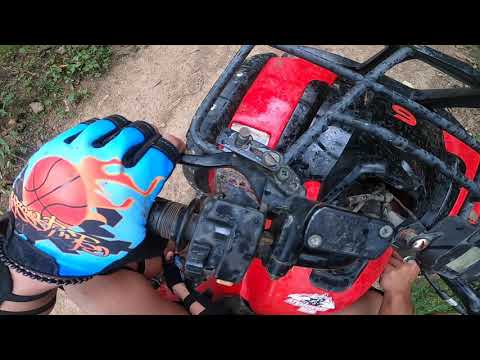The image is a top-down view of a person operating a machine, possibly a motorcycle or lawnmower. The foreground shows their left hand gripping a handlebar, adorned with a turquoise fingerless glove featuring a flaming basketball and some sort of text. The machinery itself is a mix of bright red and black parts, with the number 6 visible on a red section. In the bottom right corner, a bare Caucasian hand, potentially the person's right hand, is also touching the machine. The background consists of a beige and brown dirt path with patches of green grass and plants scattered around.